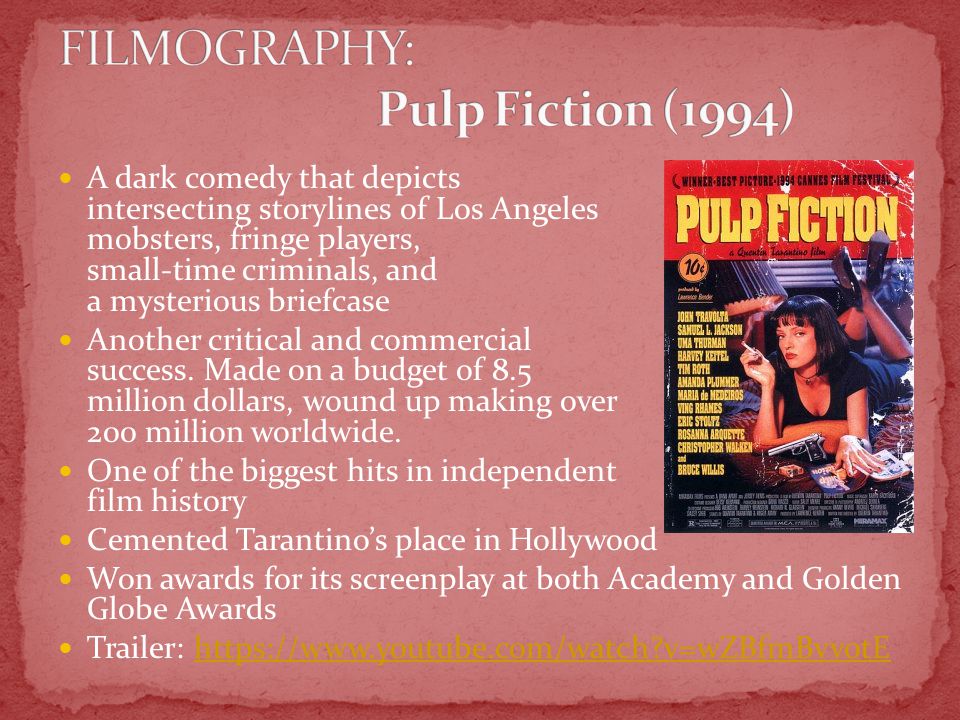The slide, resembling a PowerPoint presentation or an advertisement, provides an in-depth overview of the movie "Pulp Fiction" against a bold backdrop comprising a dark pink border and a solid pink background. Dominating the upper left corner, large all-cap white letters reading "FILMOGRAPHY:" set the stage, followed by the centered title "Pulp Fiction (1994)" in white text. The information unfolds through six left-aligned white bullet points highlighting the film's key aspects: 

1. Described as a dark comedy depicting intersecting storylines of Los Angeles mobsters, fringe players, small-time criminals, and a mysterious briefcase.
2. Noted for its critical and commercial success, made on a budget of $8.5 million and grossing over $200 million worldwide.
3. Recognized as one of the most significant hits in independent film history.
4. Credited with cementing Quentin Tarantino's place in Hollywood.
5. Awarded for its screenplay at both the Academy and Golden Globe Awards.
6. The final bullet point, in yellow text, provides an almost unreadable trailer link due to its light color against the background.

The right side of the slide showcases a vivid image of the "Pulp Fiction" cover, potentially a DVD or book cover. This iconic image features Uma Thurman lying on her stomach, clad in a short-sleeve black shirt, with short black hair. She holds a cigarette in her right hand, with a gun placed in front of her. The names of the main cast like John Travolta, Samuel L. Jackson, among others, are listed on the left side of the image, styled akin to a Pulp Fiction novel.